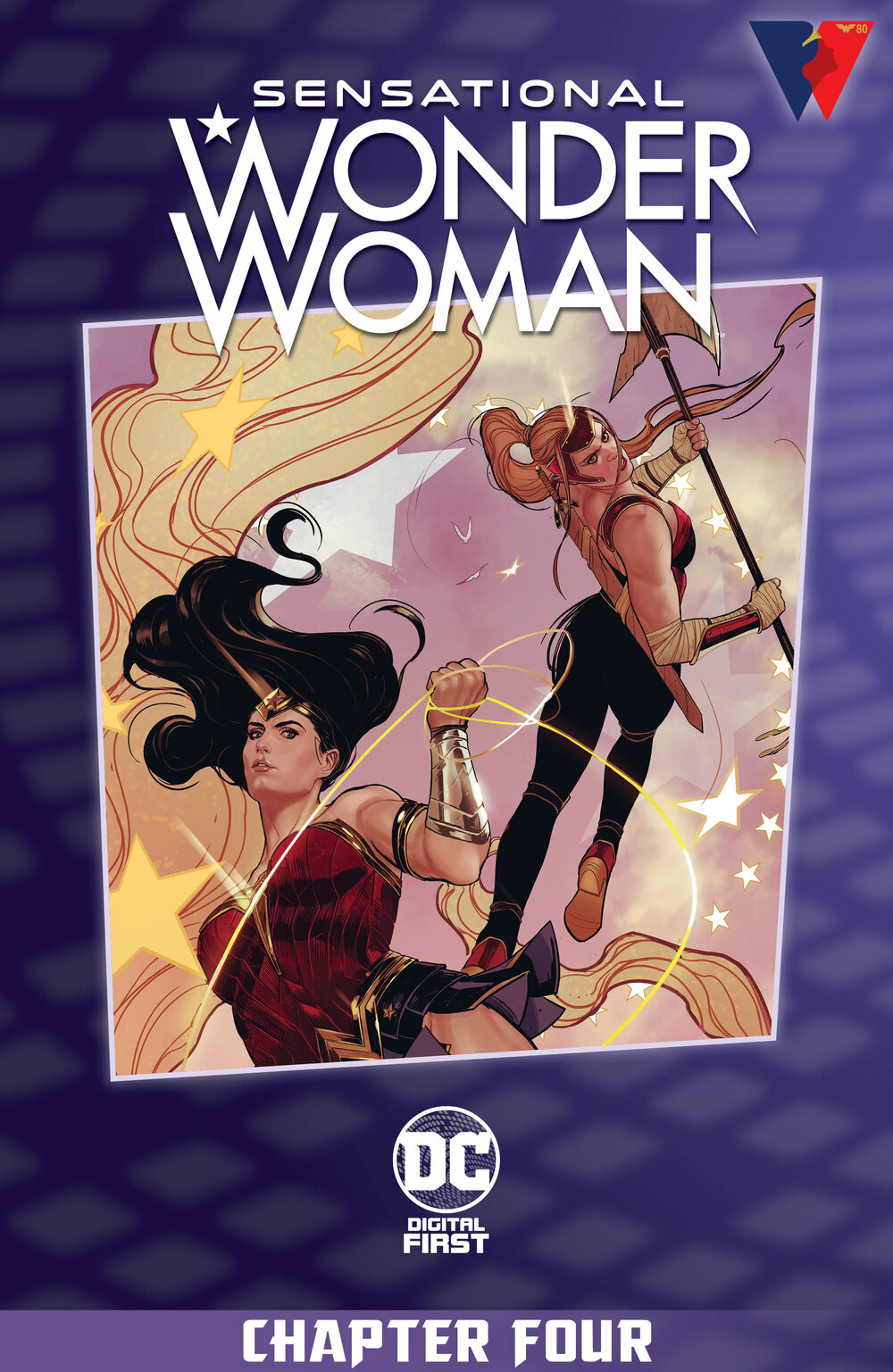This vibrant image serves as an advertisement for a comic titled "Sensational Wonder Woman," prominently featuring the iconic DC logo within a circle at the bottom. The phrase "Digital First" is displayed, followed by "Chapter 4" beneath it. In the upper right corner, a striking blue and red Wonder Woman symbol, shaped like a "W," stands out. 

At the heart of the image, Wonder Woman commands attention with her dynamic pose, her magic lasso held aloft in her upraised arm, its energy almost palpable. Her hair streams dramatically in the wind, accentuating the sense of motion and power. Behind her stands another female figure, mid-air with her back arched and a mysterious weapon in her hand, resembling a crescent moon. The interaction between the characters suggests a story brimming with action and intrigue, although the identity of the second figure remains ambiguous—whether she is an ally from Wonder Woman’s home island or a formidable foe is uncertain. 

The entire composition, rendered in an animated comic book style, encapsulates the thrilling and vibrant world of Wonder Woman, inviting readers to dive into this latest chapter of her adventures.